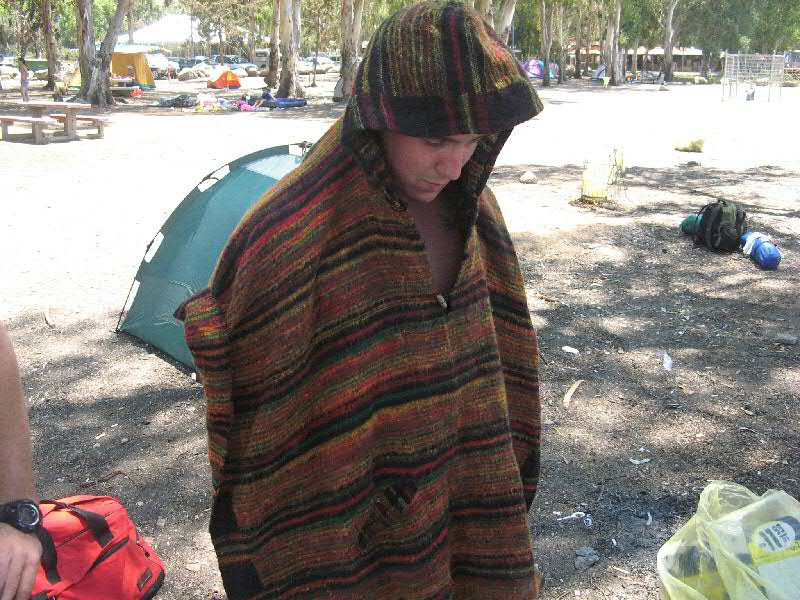In this image, we see a young man standing in a busy campground looking down at the dirt ground. The photograph is taken from a close-up perspective, capturing him from the waist up. He is wearing a thick, quilted cotton poncho adorned with horizontal stripes in colors such as brown, green, red, black, and a touch of yellow, featuring a hood and a zip-up neckline with a Mexican collar pattern. Scattered around him are various items; an orange duffel bag lies on the ground behind him, while a couple of grocery bags are seen next to him. A teal tent and picnic tables can be seen in the distance, adding to the bustling atmosphere of the recreational park. The background reveals more tents, an iron fence, benches, and a vast parking lot with several backpacks, thermos jugs, and a blue tent. A red backpack and a plastic bag, likely filled with trash, are also visible, along with a man's arm wearing a black watch. The scene depicts a lively campsite with trees, dirt, mulch, and gravel, suggesting it's a popular spot for outdoor activities and camping.